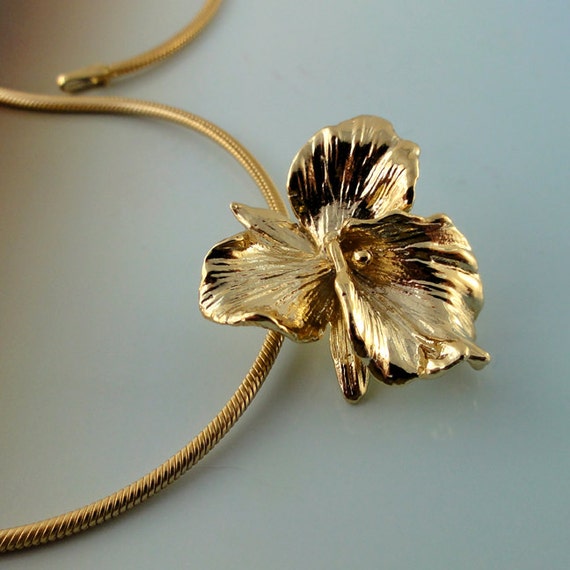The photograph features a close-up shot of a gold piece of jewelry, highlighting a pendant and its accompanying rope chain necklace. Positioned against a calm, light blue background, the focus is on the gold pendant, which resembles a flowering plant with three large, overlapping petals and two small, thin leaves beneath. The center of the flower showcases a round gold bead, adding to its detailed design. Despite the reflective, glittering nature of the gold, the pendant does not appear to be real gold but rather gold-plated. The necklace itself is a deeper gold hue, featuring a braided cable style, and we can see a portion of it along with its clasp at the top of the image. The photograph appears to be amateur in quality, indicated by its setting and angle.